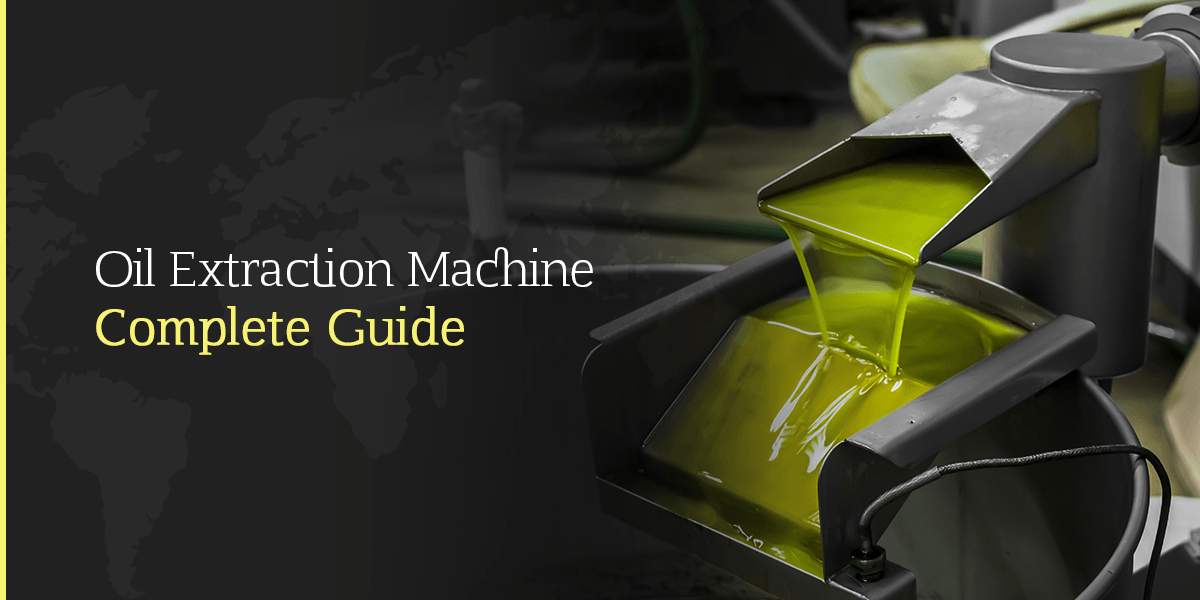The image depicts a gray metal oil extraction machine prominently positioned on the right-hand side. This machine features a flat, elongated spout from which a yellow-greenish viscous liquid, resembling fine olive oil, is pouring into a graduated tray below, eventually trickling into a larger container. On the left-hand side of the image, against a black background with faint outlines of world continents, are the words "Oil Extraction Machine" in bold white lettering and "Complete Guide" in a yellow font that complements the color of the oil. The overall design is simple yet striking, with the gray tones of the machine and background contrasting vividly with the vibrant yellow of the oil and the clear, readable text.